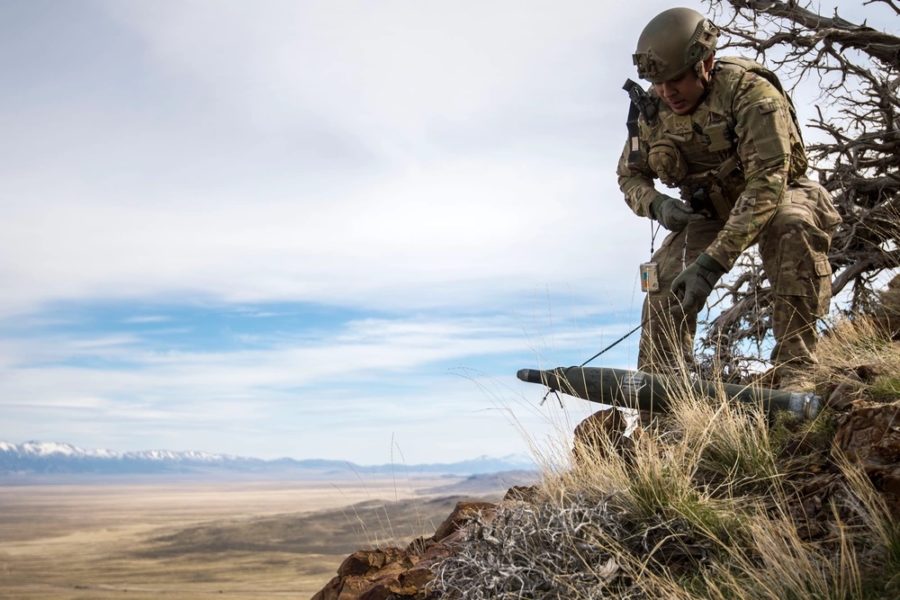In this striking image, a man, seemingly part of the American military or special operations, stands prominently on the right side of the photograph, dressed in full tactical gear. He is adorned in camouflage, with a round green helmet and dark green gloves, a long-sleeved camouflage shirt, and matching cargo pants. The man is holding a large, elongated missile-like warhead delicately by a string from its tip, suggesting it could be a potential live bomb. He stands on the edge of a cliff, maneuvering the warhead carefully over the rocky terrain. Behind him stretches a vast, barren landscape of desert with various shades of tan and brown, leading up to distant snow-capped mountains. The scene is framed by an almost surreal backdrop, where the mountains and expansive sky with scattered clouds create an almost painted effect, contrasting sharply with the realistic foreground.